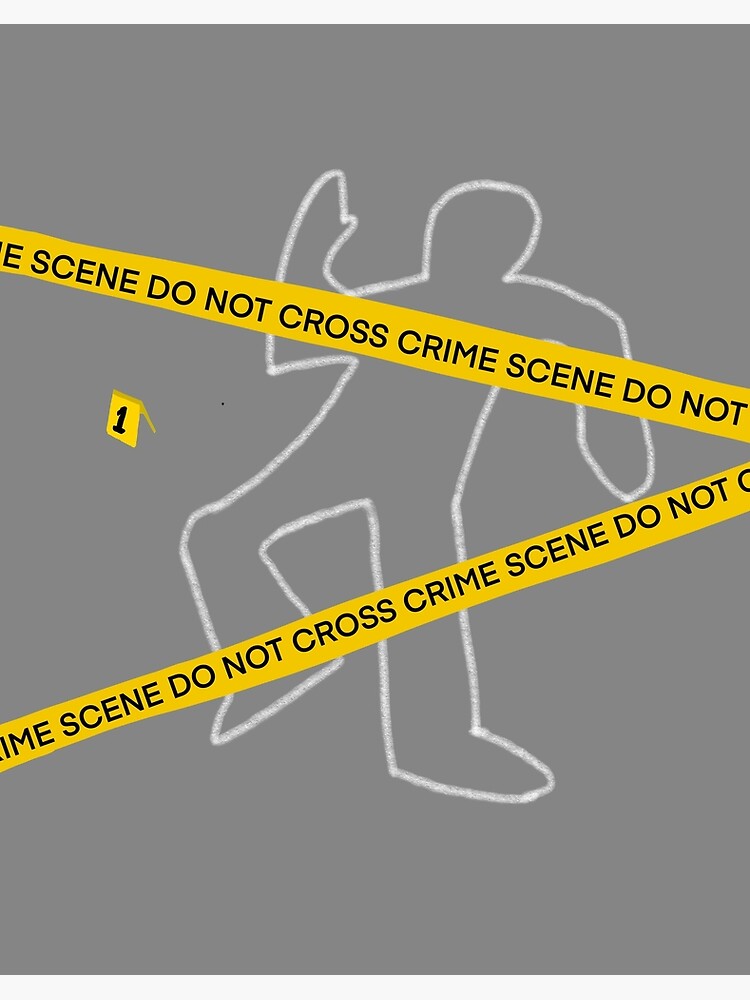The image portrays a digital representation of a crime scene on a medium slate gray background. A white chalk outline of a human figure lies flat, marked with details suggesting a victim's presumed position—left arm extended and bent at the waist, right arm reaching upwards, and right leg slightly bent. Diagonally traversing the image from the upper left to the center right, and from the bottom left to the middle right, are two vivid yellow crime scene tapes bearing the black typeset warning, "CRIME SCENE DO NOT CROSS, CRIME SCENE DO NOT." Adjacent to the chalk outline is a small yellow placard with the number "1" denoted in black. This composition captures the essence of a cordoned-off crime scene, implying efforts to preserve the area for further investigation and evidence collection by authorities.